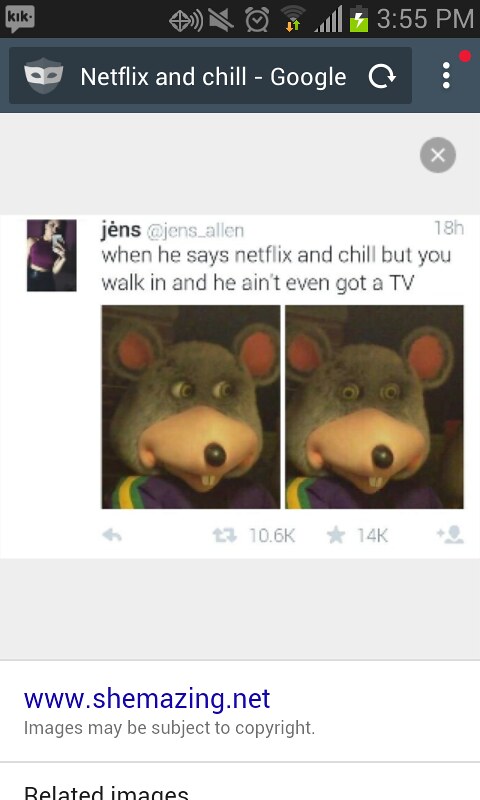This image is a detailed screenshot taken on an Android mobile device, revealing various elements on the screen. In the top left corner, notifications are visible: a Kik messaging notification, sound disabled, an alarm clock, full Wi-Fi signal, and a somewhat drained but charging battery. The time displayed is 3:55 PM. The screenshot appears to be taken within an incognito mode web browser after a search for "Netflix and chill" on Google. Below the search bar, there's an embedded screenshot likely taken from Twitter by a user named Jens (@JensAllen). The tweet humorously states, "When he says Netflix and chill, but you walk in and he ain't even got a TV," accompanied by a meme of the Chuck E. Cheese mascot looking side to side and straight ahead. Underneath the meme, there's a watermarked URL, www.sheamazing.net, followed by a section labeled "related images" in black text. The central focus of this composite screenshot is the Chuck E. Cheese meme, surrounded by the predominantly black, white, gray, green, yellow, dark blue, and maroon interface, emphasizing that the entire scene is a smartphone capture.